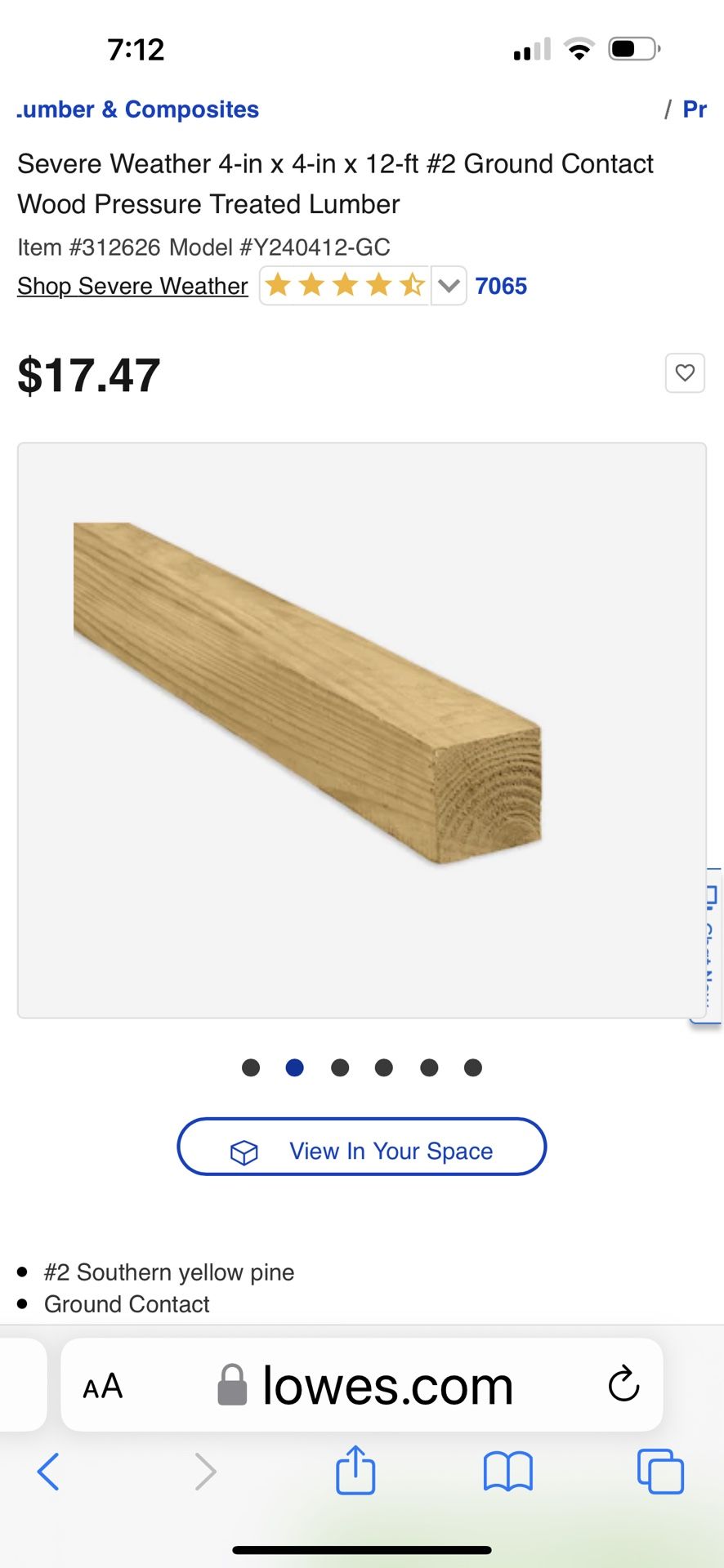In the upper section of the image, the background is white, displaying the time "7:12" in black on the left-hand side. Below the time, partially cut off, is the text "U-N-B-E-R" in blue with the symbol for capacitance. Following this, in black text, is the phrase "Severe Weather" with "4-IN" (indicating 4 inches) and "X 4-IN". Next to this is "12-FT" (indicating 12 feet), and "#2 ground contact." 

Further down, still in black text, the image reads "Wood Pressure Treated Lumber." Below this, it mentions "Item #312626" and "Model #Y240412GC”. Under a line, the text "Sharp Severe Weather" appears. There are approximately 1.5 stars displayed, suggesting a low rating, with the number "7,765" in blue indicating the number of ratings. The price is listed as "$17.47" in black text.

The lower section of the image shows a gray background with a beige wooden plank. An oval outlined and filled in blue contains the text "View In Your Space." Below this are two bullet points in black: the first reads "#2 Southern Yellow Pine," and the second indicates "ground contact."